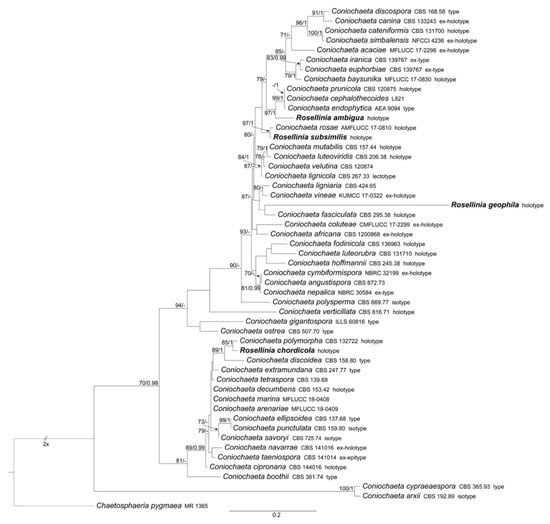The image is a detailed graphical representation of a biological divergence tree, starting from the lower left and branching out towards the top right. It features approximately 50 genus and species names, all italicized, with some in bold font like Rosalina ambigua, Rosalina similis, Rosalina genophila, and Rosamelia corticola. The entire chart is set against a solid white background, with lines (acting as brackets) connecting the names in a descending, concave manner, illustrating their hierarchical relationships. At the top of the tree is Coniochaeta discospora, and the structure becomes more complex towards the bottom as additional branches form. This diagram serves as a scientific categorization, likely in Latin, detailing different biological classifications. There are no pictures, only black text on a white background.